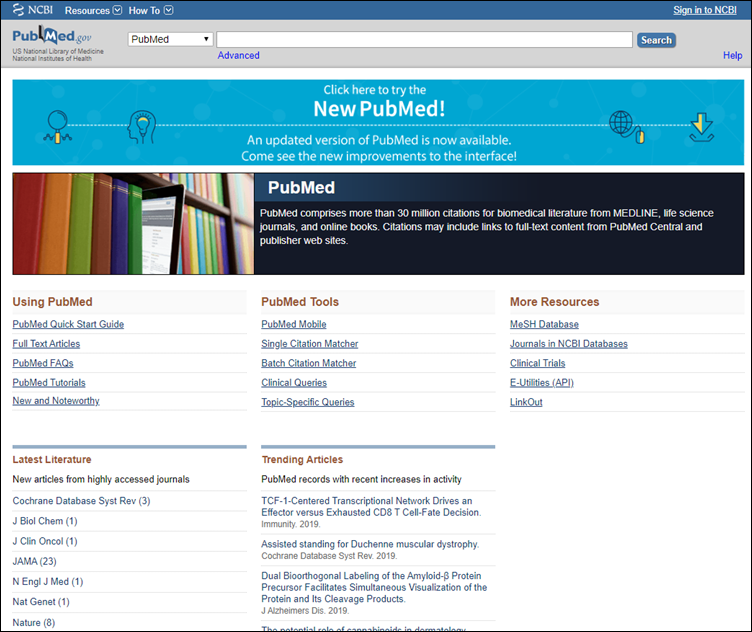The image is a screenshot of the NCBI website, highlighting its main section. At the top, there is a prominent, thick banner stretching horizontally across the page. In the center of this banner, a clickable prompt reads, "Click here to try the new PubMed." To the left of this banner, a series of interconnected icons is depicted: it begins with a round symbol, followed by a line leading to a head with a lightbulb in the middle, signaling innovation or ideas. This line continues through the center to an earth symbol, representing global access or reach, and finally connects to an arrow pointing downwards, suggesting an actionable step or download. Below this line, a message invites users to "come see the new improvements to the interface."

Directly beneath this banner, and separated by some space, is another section designed like a bookshelf filled with books. A tablet is partially protruding from the shelf, its corner visible. To the right of this visual arrangement, the word "PubMed" is prominently displayed, followed by a brief description or blurb regarding PubMed.